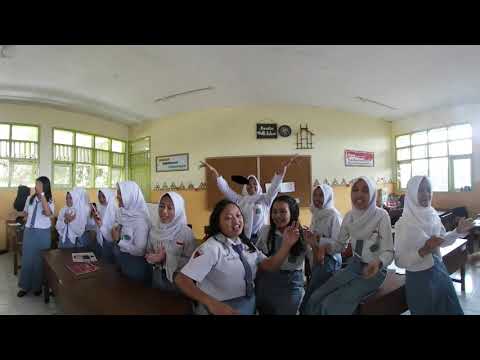This image captures a vibrant classroom scene with perhaps 15 young Asian women who appear to be high school-aged. The majority of the women are dressed in white blouses paired with white headscarves, giving a cohesive and uniform appearance. Among them, three girls stand out as they do not wear the white headdresses; instead, they are dressed in white tops and blue dresses. The room's walls are painted yellow and the ceiling white, creating a bright atmosphere enhanced by sunlight streaming through the windows on the left and right sides. Brown wooden desks are scattered throughout the room, with some pushed together to form clusters where the girls are seated closely. At the center of the scene stands a striking figure: a woman possibly in an official capacity—maybe police or military—distinguished by her green tie and light-colored shirt. Behind her, another woman with raised hands, possibly singing into a microphone, adds dynamism to the tableau. The overall scene is slightly distorted due to the photograph being taken with a GoPro, giving the yellow back wall a curved appearance.